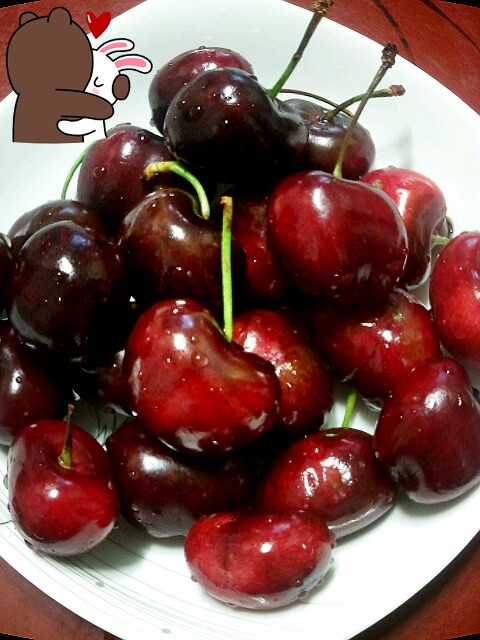This close-up photograph features a rounded square white plate, possibly adorned with some fine silver bordering or light scratch markings. The plate is piled with approximately 20 to 25 ripe cherries, varying in shades from deep red to almost dark purple. Each cherry has a green or brown stem, and water droplets cling to their freshly washed, glistening surfaces. In the upper left corner, there is a whimsical, semi-transparent cartoon logo showing a brown bear hugging a pink and white rabbit with a small red heart floating above them. The background hints at a light reddish-brown table with some black lines visible in the top right corner.